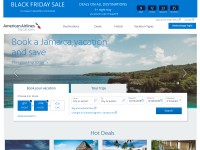The image appears to be a blurry screenshot divided into multiple sections highlighting a promotional advertisement. 

At the top inch of the image, the background is a dark blue, and in the left corner, there is large white text in all capital letters reading “FRIDAY'S BLACK FRIDAY SALE.” Underneath, there is some smaller white text that is too blurry to decipher. 

In the center section, three rows of white text are present but illegible due to the blurriness. On the right side of this section, there are three to four black squares containing gray letters and white text underneath, neither of which can be made out clearly.

An approximate one-inch white border follows. Within this border, “American Airlines” is written in black text. Four additional black words are present but unclear. On the right side of this boundary, there is a blue tab with some white lettering that is also indiscernible.

Below, there is a larger photo taking up about two-thirds of the image height, extending down to about two inches from the bottom. A pop-up tab overlays part of this photo at the bottom edge. In the top left corner of the photo, the blue text reads, “Book a Jamaican vacation,” followed by, “and save” in blue right below it.

The photo shows a landscape with a cloudy sky on the left side, water below it, and green grass occupying the right side, the scene almost perfectly divided between the water and grass. A white pop-up tab spans almost the entire width of the image, containing three squares (two blue ones and one white), filled with more indiscernible information.

On the far right of the photo, another blue tab with white text is visible. Below this, the phrase “Hot Deals” is centrally located at the bottom of the image. The very bottom edge captures the top portions of four additional pictures.